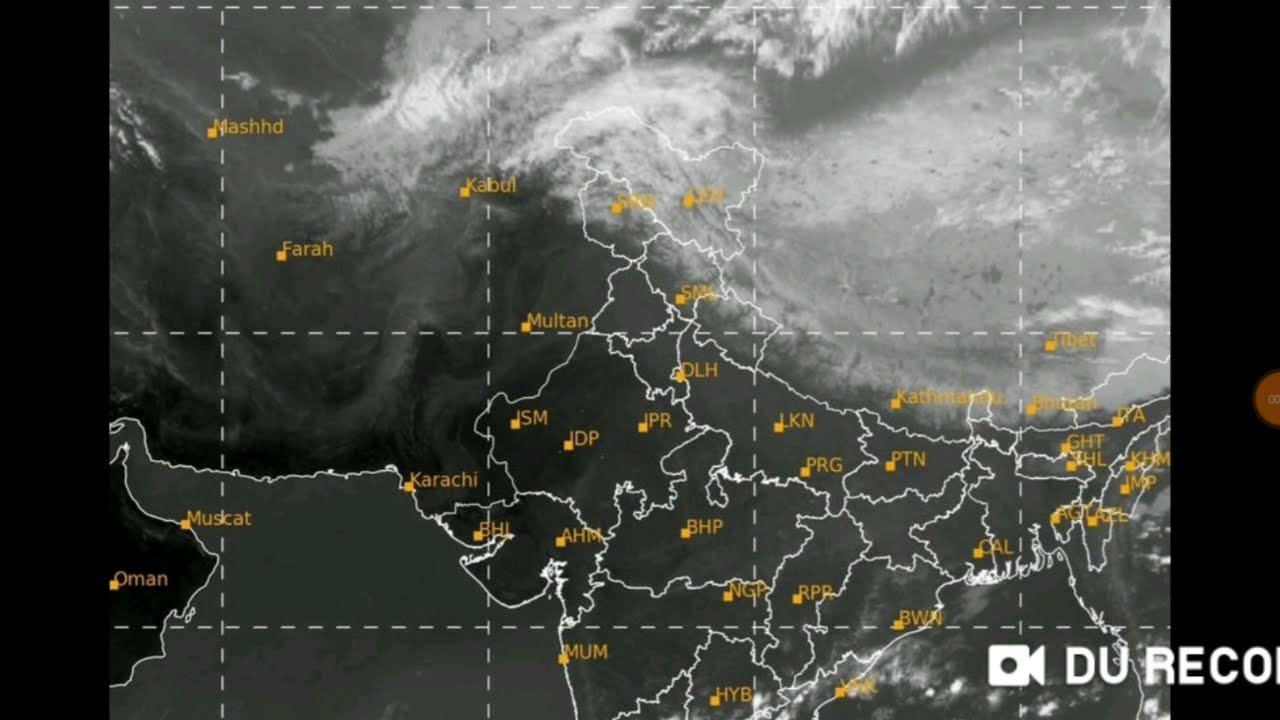The image is a satellite view of a portion of the Earth, presented in black and white. The land is divided by a rectangular grid of dashed gray lines, forming a matrix of approximately three rows by four columns. The terrain includes mountainous regions with cloud cover, and a body of water is visible in the lower left corner. Various locations are marked with small yellow squares, labeled with either full names like Mashd, Farah, Kabul, Multan, or three-letter abbreviations such as ISM, IDP, IPR, and DLH. These labels appear in orange text. In the lower right corner of the image, a video camera icon and the text "DU RECO" are visible, suggesting a video format. The overall view is a top-down perspective, capturing detailed geographical boundaries and weather conditions affecting the area.